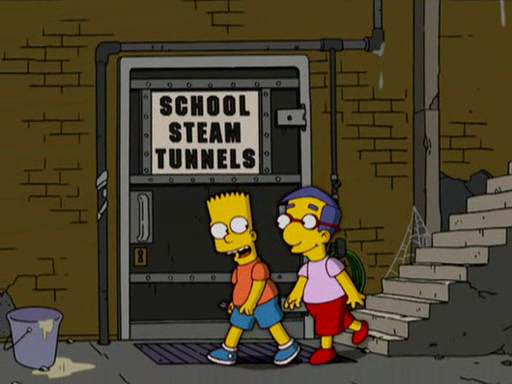This image captures a moment from The Simpsons, featuring Bart Simpson and his friend Milhouse descending a set of stairs outdoors. Behind them is a brown brick wall with visible water pipes and a metal door labeled "School Steam Tunnels" in black text on a white background. Bart, known for his yellow skin and spiky hair, is donning his usual orange short-sleeved shirt, blue shorts, and blue sneakers. Milhouse, recognizable by his purple hair, red glasses, and lavender t-shirt, is wearing red shorts and red sneakers. They are walking to the left of the image, and Bart appears to be saying something to Milhouse. In front of them, at the base of the stairs, there's a purple bucket with water spilled onto the concrete floor and a small drip hanging from its lip. A welcome mat lies near the door, and a spider web can be seen next to a cement column extending upwards along the brick wall.